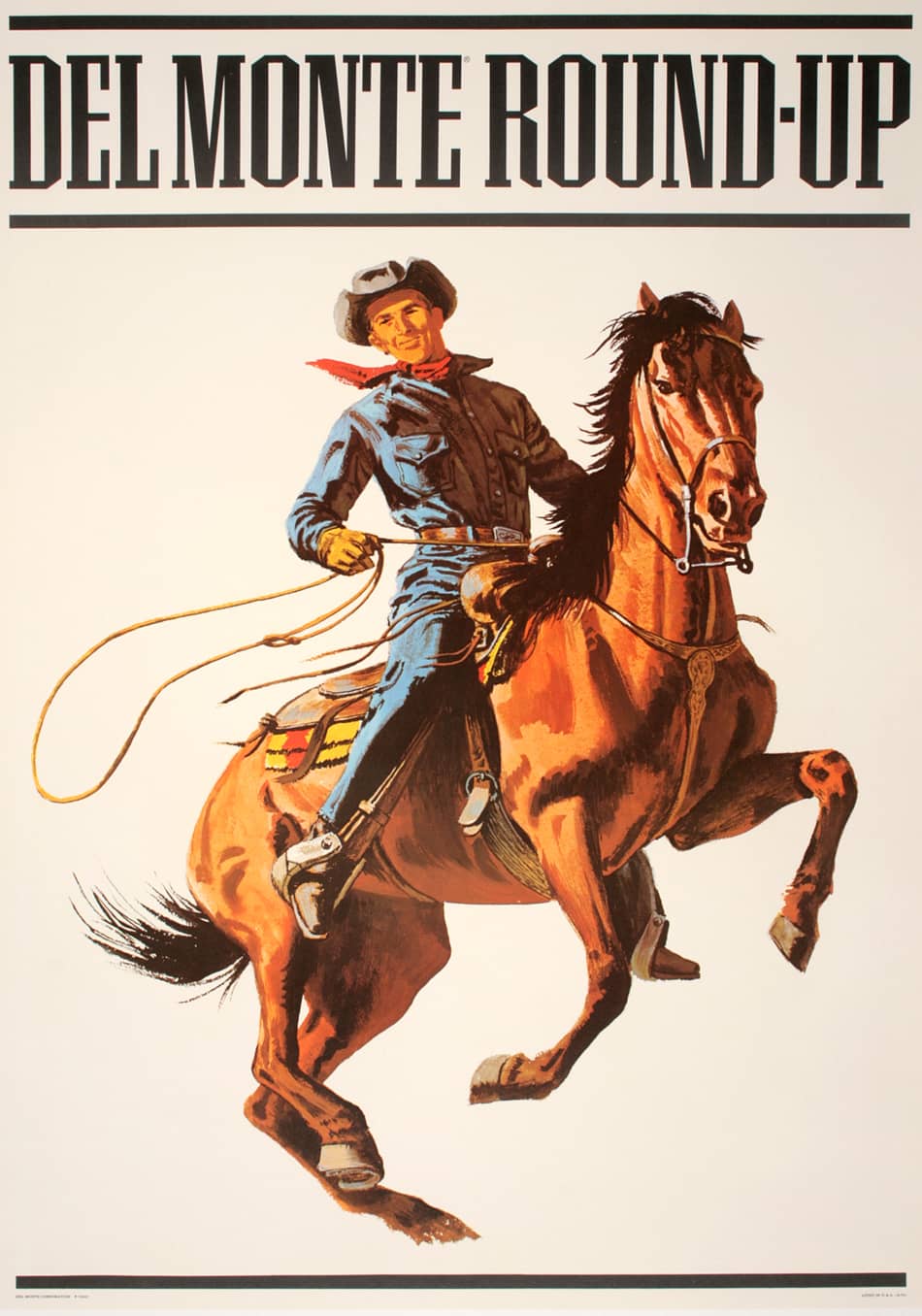This vintage-style advertisement features a vibrant illustration of a cowboy riding a rearing brown horse with a black mane and tail. At the top of the image, in bold black letters, it reads "Del Monte Roundup," set against a gray background with black stripes above and below the text. The cowboy, dressed in denim pants and shirt, a gray hat, a red bandana around his neck, and a brown belt, confidently holds a lasso in his right hand. The horse is equipped with a brown saddle and a reddish-yellow blanket underneath, with the cowboy's feet secured in the stirrups. The pale-colored background enhances the nostalgic, old-school feel of this striking Western-themed poster.